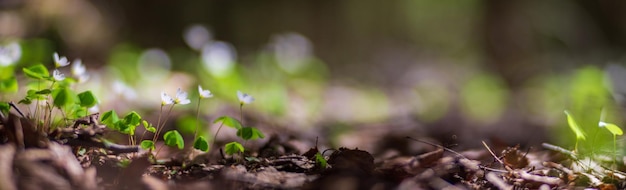This close-up, horizontally elongated photograph captures a ground-level view of a natural scene. The bottom portion of the image shows a dirt-covered ground scattered with brown, dry leaves. Among the leaves, on the left side, small green plants are emerging, each bearing 2-3 leaves and a single white flower at the top. There are about 7-8 such plants clustered together. The photograph was taken outdoors during the daytime, with the background intentionally blurred, revealing hints of brown, green, and white colors. The blurred section occupies the top part of the image, enhancing the focus on the intricate details of the ground-level flora.